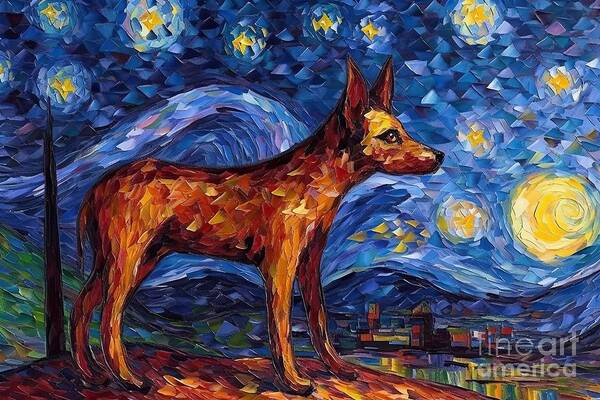The image depicts a detailed painting or collage of a brown dog with pointed ears, composed of various geometric shapes such as triangles and trapezoids. The dog stands on all four legs atop a brown mount, appearing to gaze to the right. The piece is rectangular, with the top and bottom sides being twice as long as the left and right sides. The background is reminiscent of Van Gogh's style, specifically "Starry Night," featuring a blue sky adorned with swirling yellow circles, and created with small triangles of different blue hues. Beneath this vivid sky, a distant town near a lake can be seen, its reflection capturing the sky's colors in a smudged, abstract manner. The scene includes a black pointed spike in the distance, adding to the complexity of the composition. In the bottom right corner of the painting, a semi-transparent white watermark reads "fine art" on the top line and "america" on the bottom line, both in lowercase letters. This meticulous and vibrant artwork skillfully blends impressionistic styling with geometric precision.